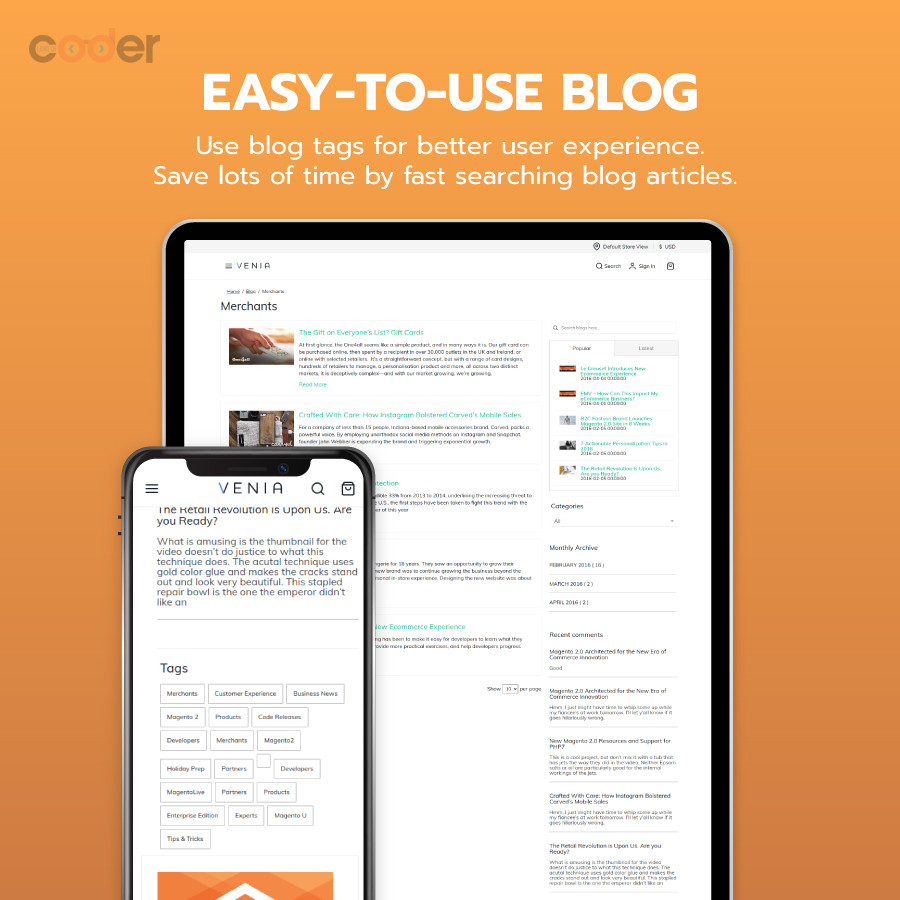The image features a smartphone and a tablet against an orange background. In the upper left corner, the word "Coda" is written in a combination of brown and orange. At the top center, prominent white text reads "Easy to Use Blog," with smaller white text below that states, "Use blog tags for better user experience. Save lots of time by fast searching blog articles."

The tablet is positioned behind the smartphone, displaying two images accompanied by several paragraphs of text. The text has blue headlines, while the main content is written in black. On the smartphone screen, the word "Venia," spelled "v-e-n-i-a," is prominently displayed in black. Below this, a paragraph of text is visible, along with several rectangular tags, providing a seamless browsing experience.

This layout emphasizes the ease of navigation and efficiency offered by using blog tags for a better user experience on digital devices.